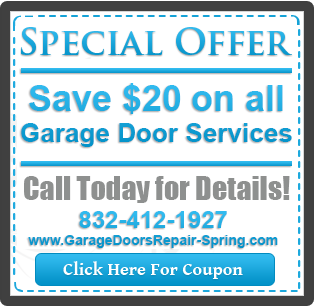This image showcases a digital coupon offer typically found on websites. The coupon is square-shaped with a black border and a white background. At the top, bold black text announces "Special Offer - Save $20 on all garage door services." Directly below, in smaller gray text, it reads, "Call today for details," accompanied by the phone number 832-412-1927. Further down, the website address "garagedoorsrepairspring.com" is displayed. At the bottom, a blue rectangular button with white text invites users with a prompt: "Click here for coupon." The design suggests that this offer is meant to attract potential customers through online advertisements.